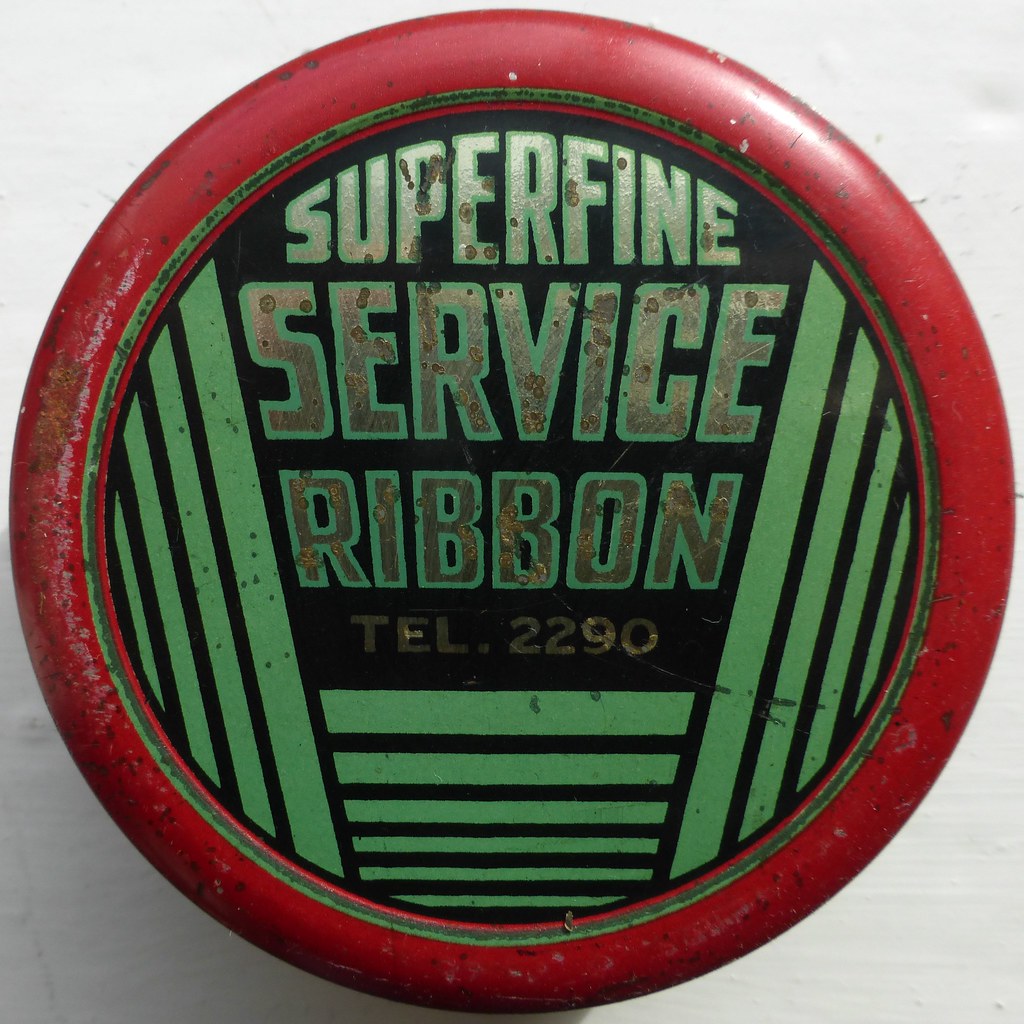The image depicts a worn, circular object that appears to be either a logo, pin, or possibly a cap for a container. The object has a red, round border, showing signs of age and wear with scratches, dirt, and some rust. The center features a dark background with green and black stripes, where the horizontal lines are intersected by angled, vertical lines. The text "Superfine Service Ribbon TEL 2290" is inscribed in silvery letters, possibly chipped or partially covered by paint, adding to its old and used appearance.